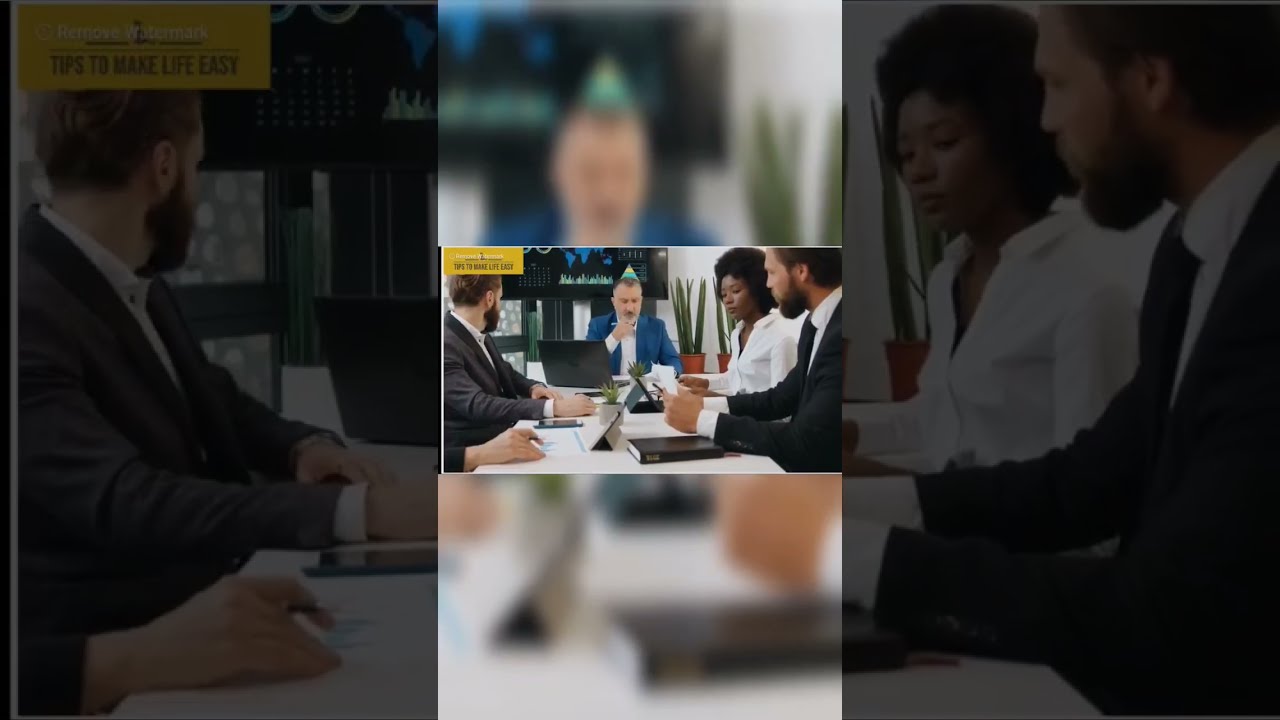The image is a composite photograph, with a central, detailed picture of a business meeting surrounded by blurry, faded, geometrically-sectioned versions of the same photo. In the main image, four people are seated at a white conference table, which is cluttered with books, papers, and a laptop, with other attendees using tablets. The focal point is an older Caucasian man seated at the far end of the table, leading the meeting. He is wearing a blue suit jacket over a white button-up shirt, without a tie, and has short hair and a beard. To his right sits an African American woman with short, natural hair, clad in a white blouse, and next to her is a Caucasian man in a gray suit with a brown beard. Across the table is another Caucasian man with short brown hair and a beard, dressed in a dark gray suit. Partially obscured hands suggest the presence of a fifth person. Behind the leading man, a TV screen is visible. The primary image is set against a backdrop that consists of the same photograph, enlarged and blurred, serving to frame and accentuate the central scene.